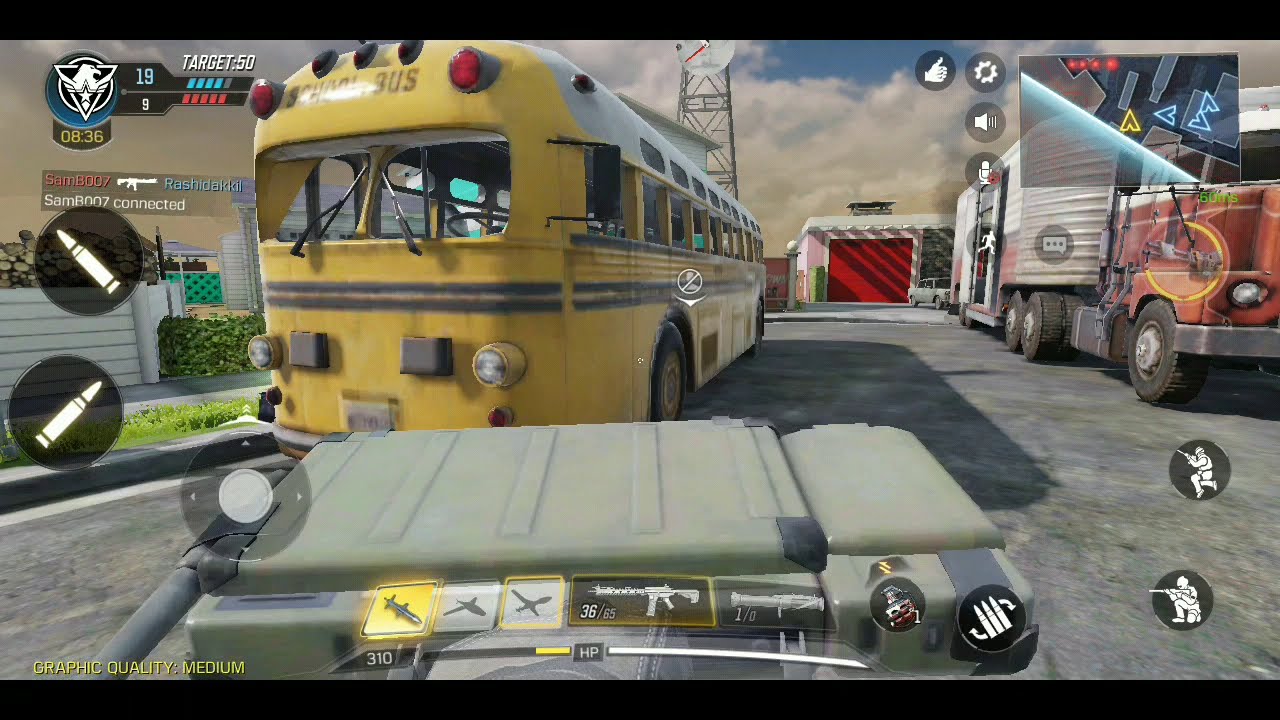This detailed scene from a first-person shooter video game features a vibrant, albeit slightly cartoony, environment. The centerpiece is a yellow school bus positioned on the left side of a wide gray asphalt road, displaying black stripes along its faded sides and notable red headlights at the front. A green rectangular object, possibly a military-style ammo storage container or cooler, is immediately in the foreground, indicating it might be actively engaged with or opened by the player character.

To the right of the school bus stands a substantial red-fronted tractor-trailer with a rusty, reddish-brown hue, complemented by black tires and a white ridged back. This vehicle is parked on a spacious road, flanked by a sidewalk with green grass, a white fence, and a green bush on the left, leading up to a building with a red garage door in the background.

The game’s user interface (UI) is comprehensive: the upper left corner of the screen shows a score of 19 above a score of 9, with a target score of 50 prominently displayed. Below this are bullet icons and health bars. The weapon selection spans across the bottom center of the screen, while the mini-map occupies the top right corner. Various other game-specific icons fill the screen, enhancing the immersive gaming experience.